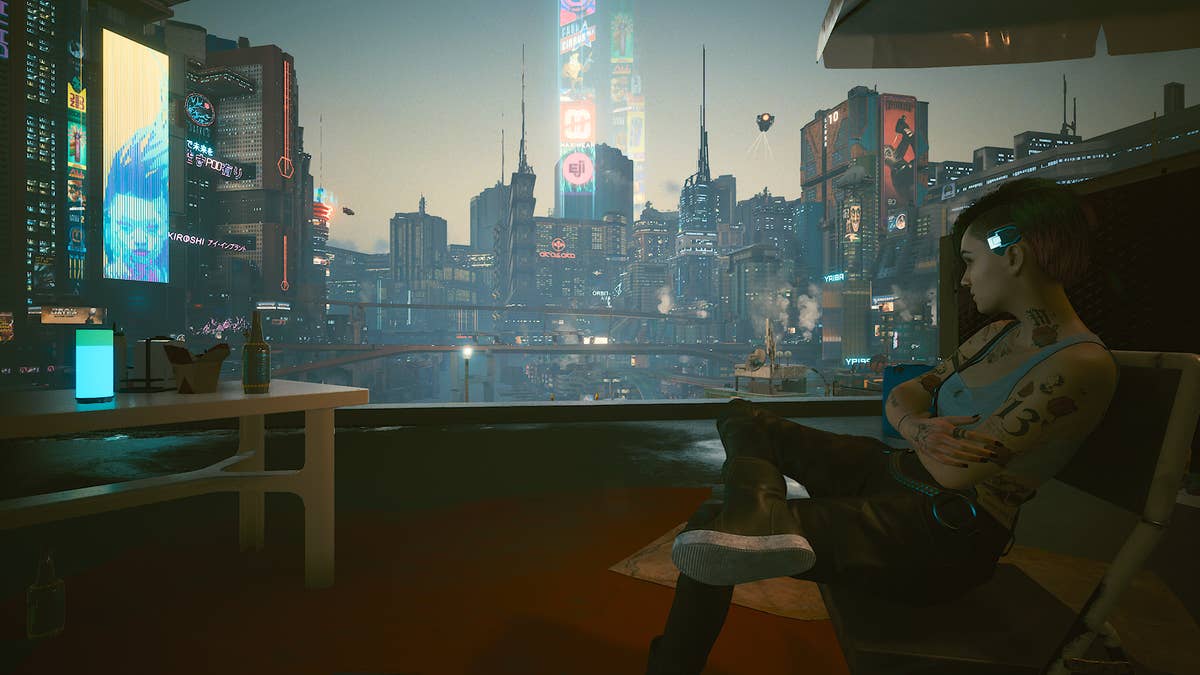The image appears to be a highly realistic computer-generated scene, potentially from a futuristic game or design project. Dominated by a panoramic glass wall, it opens up to a congested skyline bursting with towering skyscrapers, neon lights, and advertisements. Hovering vehicles or spaceships drift through the air, adding to the city's advanced, bustling atmosphere. Inside the room, a girl with tattoos, including a prominent '13' on her arm, sits pensively on an uncomfortable metal chair. She wears a gray tank top, dark pants, and dark shoes. A glowy device is affixed near her ear, enhancing the futuristic vibe. To her left stands a simple white coffee table bearing a bottle of beer and a small lit night lamp. Above the table, there's a screen—its position unclear—completing the meticulously detailed scene.